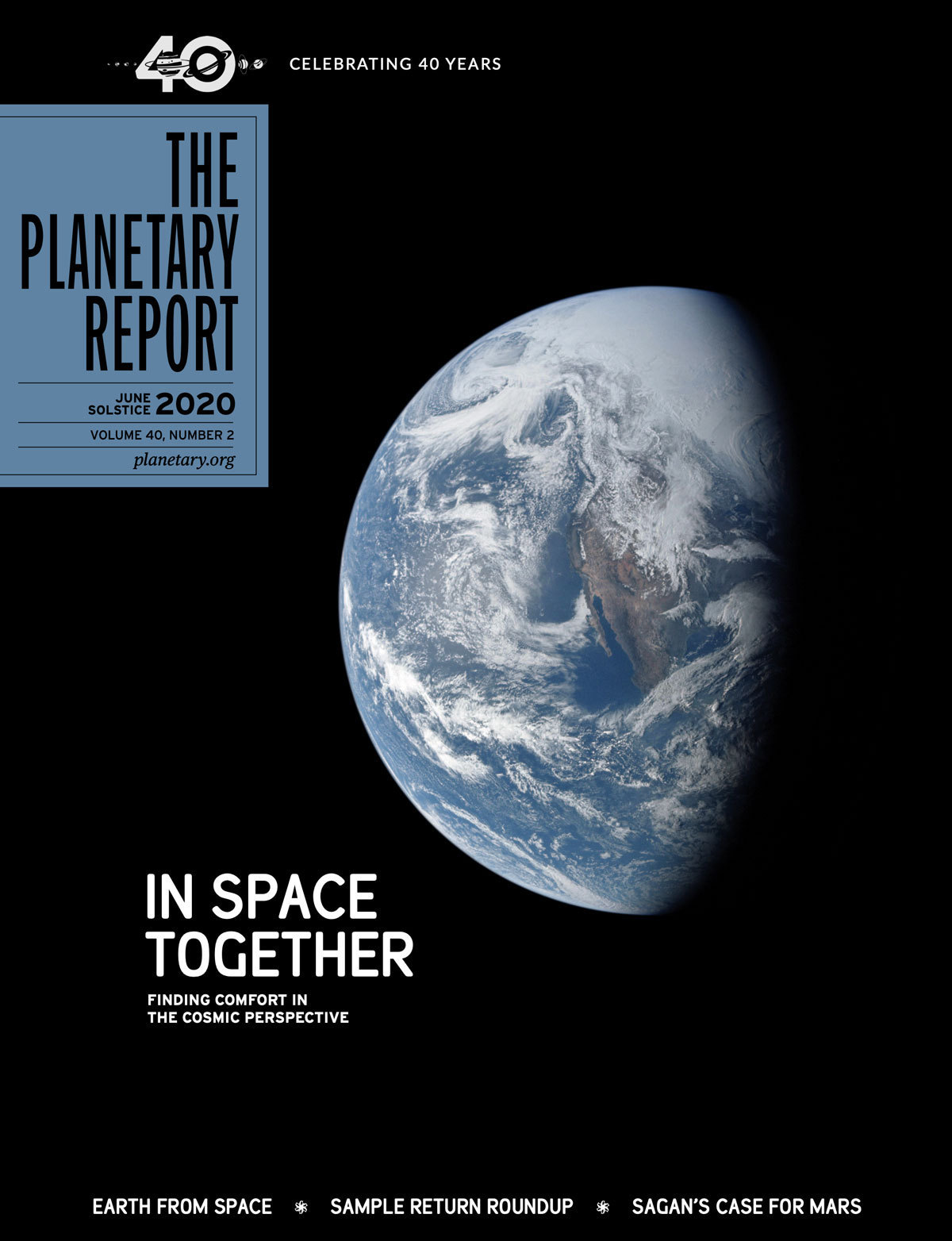This captivating image features a stunning visual of a planet set against a pitch-black background, likely representing the vast expanses of outer space. The image appears to capture Earth as seen from space, with the visible portion illuminated, showcasing intricate clouds swirling above vast bodies of water and distinct landmasses. The northernmost region is adorned with icy expanses, presumed to be the North Pole.

The text overlay is meticulously presented, celebrating four decades of cosmic exploration and insight. It reads, "40, celebrating 40 years, the planetary report, June solstice 2020, volume 40, number two, planetary.org." Beneath this, a poignant message reinforces the theme of unity and curiosity: "In space together, finding comfort in the cosmic perspective. Earth from space, sample return roundup, Sagan's case for Mars."

The layout is both elegant and thought-provoking, with the text predominantly centered to the right, harmoniously balancing the magnificent planetary portrait. The interplay of text and imagery invites viewers to reflect on our place in the universe, marking a milestone in planetary exploration and scientific discovery.